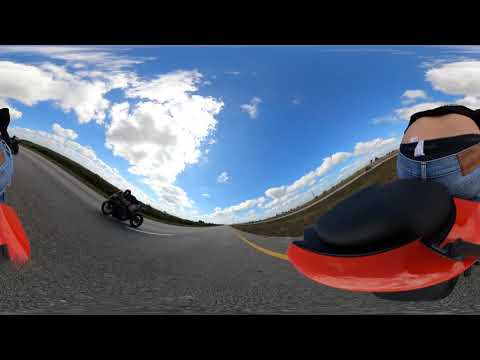The image is a somewhat distorted, low-resolution outdoor photograph, likely taken with a 360-degree or concave lens, which creates a warped effect. In the image, at least one person is riding a black motorcycle on a road that curves unnaturally due to the lens distortion. The road, which features a yellow stripe down the middle, stretches across the image and appears to tilt up to the left and down to the right. 

To the left-center of the image, there's another person, possibly a woman with long hair, standing on the road, wearing a blue top. A red object is seen hanging from her waist, however, the details are unclear due to the resolution. 

On the right side of the image, prominently visible is a person bending over a large red and black part of a motorcycle. This person’s upper body and back are partly exposed; they're wearing blue jeans with a label visible and black underwear peeking out above the jeans waistband. Their black shirt has ridden up, revealing part of their lower back.

Flanking the road are green fields under a bright blue sky filled with several large, fluffy white clouds, suggesting a sunny daytime setting. Despite the distortion, the general scene portrays a rural road and a couple of motorcyclists.